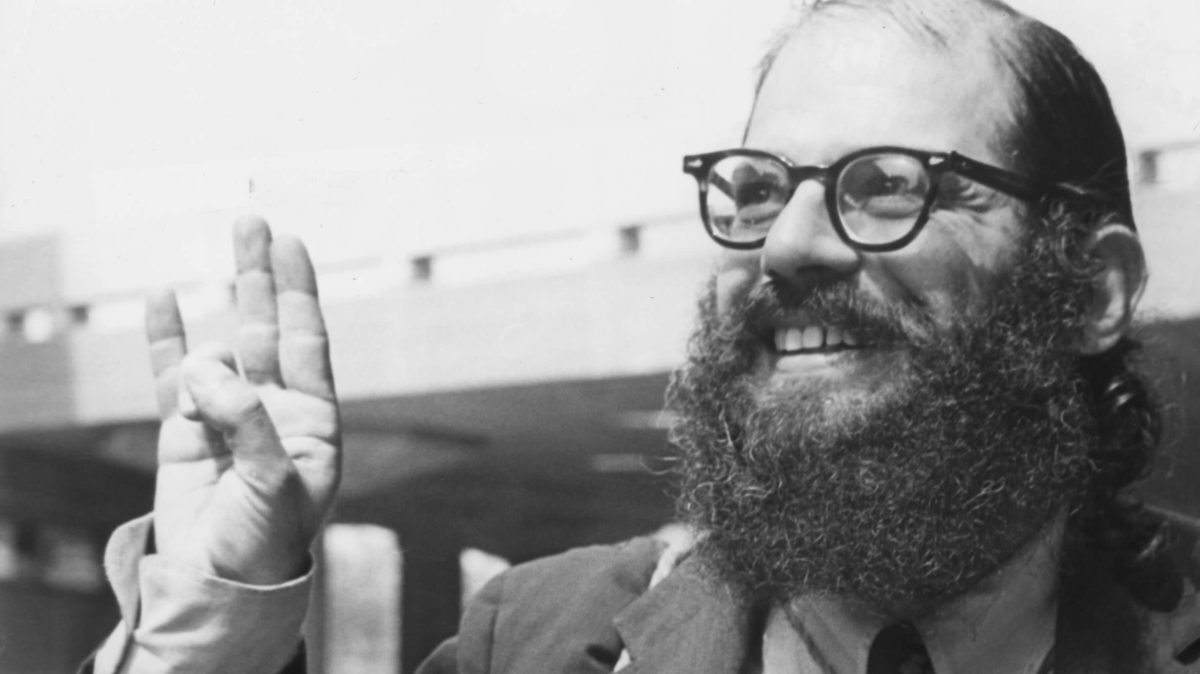In this black and white photograph, a middle-aged man, possibly in his early to mid-40s, is captured in a moment of joy. He has a full beard and wears glasses, suggesting a distinguished, perhaps scholarly, appearance. The man, likely of Jewish descent, is smiling broadly and looking off to the side, his gaze fixed on something that evidently brings him happiness. He is dressed in a suit with a vest, hinting at a professional or formal context, perhaps from the 1970s or 1980s given the image's aesthetic. His right hand is raised, forming a W-like hand sign where three fingers are extended, and his thumb touches his index finger. In the blurred background, there's an indistinct structure that could be a bridge or another architectural feature, adding a layer of intrigue to the setting of the photograph. Overall, the man exudes a sense of contentment and positivity.